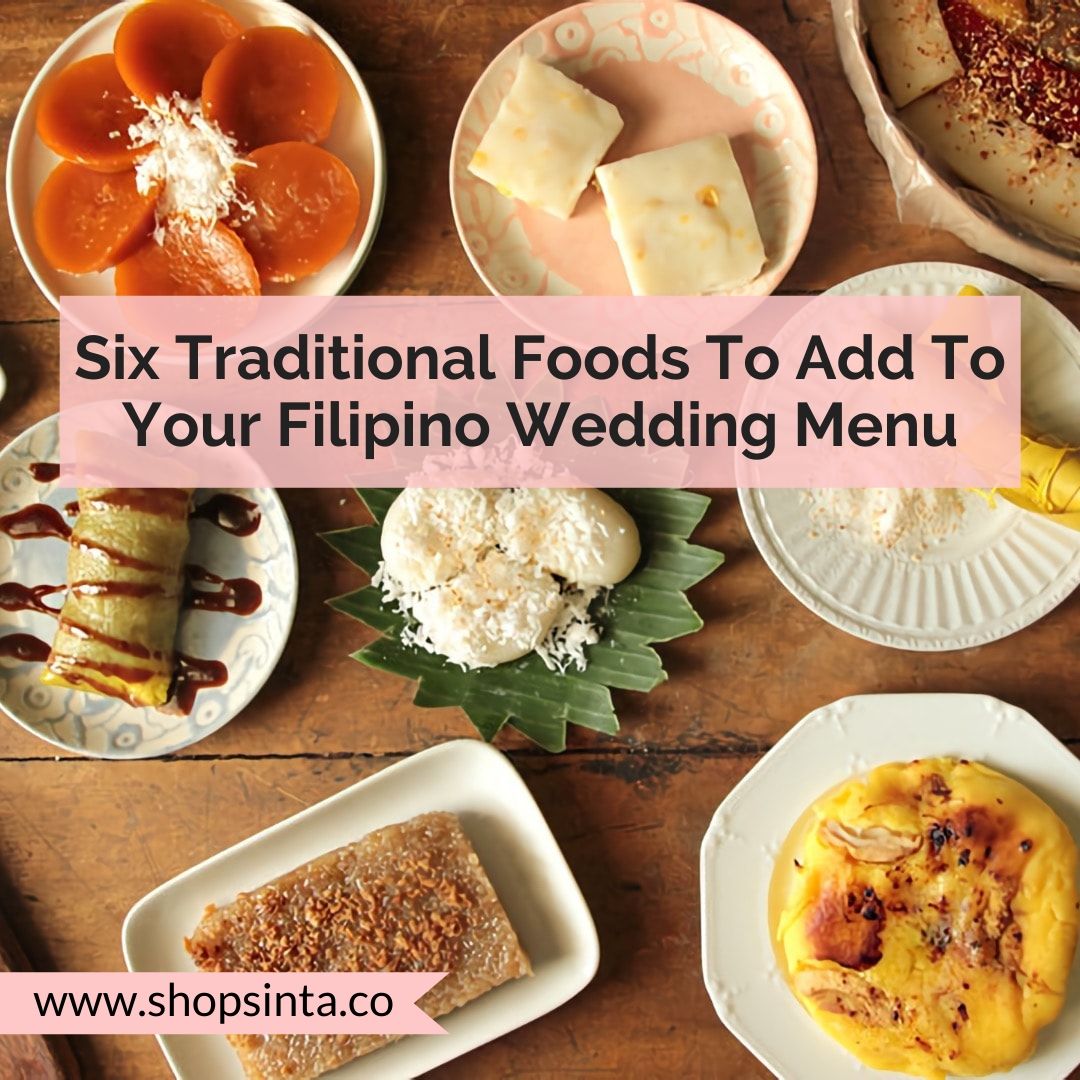The image is an advertisement for ShopCinta.co, promoting "6 Traditional Foods to Add to Your Filipino Wedding Menu." The aerial shot encompasses a rustic, slightly damaged wooden table with horizontally aligned planks, decked with an eclectic array of small, mismatched plates. These dishes vary in shapes and colors, from circular and rectangular to octagonal, each adorned with vibrant Filipino foods.

In the top center, a pink rectangle showcases the ad's title in bold black text: "Six Traditional Foods to Add to Your Filipino Wedding Menu." A similar pink banner in the bottom-left corner features the website address, www.shopcinta.co, with a distinctive forked end.

The plates, mostly saucer-sized, flaunt an assortment of appetizing items. Noteworthy dishes include:
- A green leaf with sawtooth edges serving a white, crumbly coconut-like substance.
- A white plate with circular brown vegetables sprinkled with cheese.
- A pink and white plate presenting two cream-colored squares.
- A blue and white dish featuring a sausage roll-like item drizzled with chocolate.
- An octagonal white plate with etchings, holding a bagel-like item adorned with various ingredients.
- A tan plate partially visible in the top right, suggesting an ambient rustic elegance.

These vibrant and varied dishes offer a delightful spectrum of colors and textures, embodying traditional yet visually appealing elements suitable for a Filipino wedding feast.